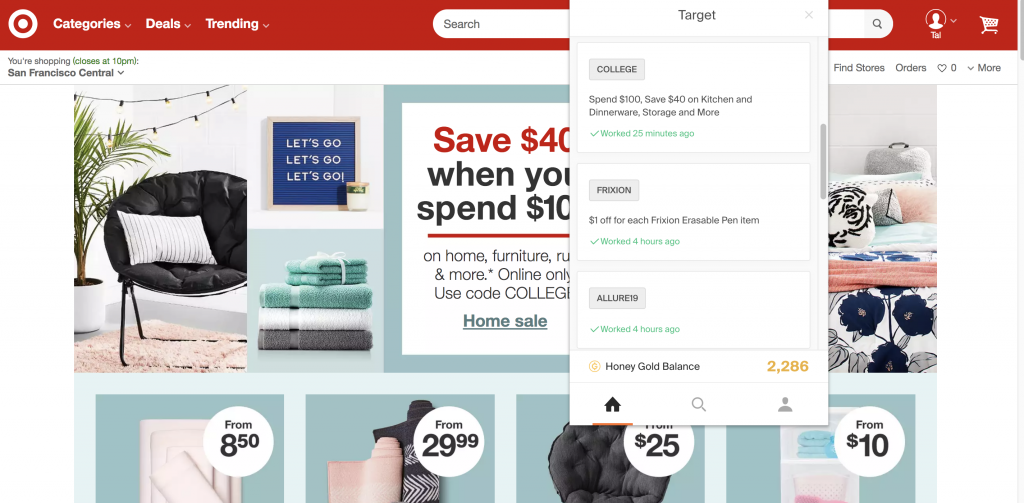A screenshot of the Target website is displayed. At the top of the page, a distinctive red banner stretches across, adorned on the far left with the recognizable Target logo. Adjacent to the logo, three menu options—'Categories', 'Deals', and 'Trending'—are presented in white font. Positioned centrally within the banner, a white search field stands out, while on the far right, white icons for account access and the shopping cart are clearly visible. Slightly overlapping the search field, a mini menu prominently displays the word "Target" at the top, followed by a small box labeled "College". The two subsequent small boxes beneath are not legible. Below this drop-down menu, the website layout features a series of photographs showcasing various products: a set of chairs, some towels, and a stylishly accessorized bedroom. A promotional banner interspersed among these images advertises a savings of $40, highlighting the offer "Spend $10 to save $40" with the numeral "40" rendered in standout red font, while the remainder of the text is in black.